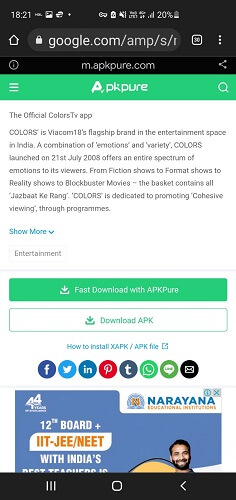A screenshot of a cellphone displays a webpage. At the top of the screen, the time is 18:21 and the battery level is at 20%. A series of icons are situated between the time and battery indicator. Below, there is a home button next to a locked padlock icon, with a URL that begins "google.com/amp/i/" but is cut off.

Further down, there is a prominent green rectangular header spanning the full width of the screen, containing the text "APKPURE". Beneath this header lies a paragraph describing the "official Colors TV app," stating in capital letters: "COLORS IS VIACOM 18'S FLAGSHIP BRAND IN THE ENTERTAINMENT SPACE IN INDIA, A COMBINATION OF 'EMOTIONS' AND 'VARIETY.'" The description continues in all capital letters: "COLORS LAUNCHED ON 21ST JULY 2008 OFFERS AN ENTIRE SPECTRUM OF EMOTIONS TO ITS VIEWERS FROM FICTION SHOWS TO FORMAT SHOWS TO REALITY SHOWS TO BLOCKBUSTER MOVIES. THE BASKET CONTAINS A DIVERSE RANGE OF PROGRAMMING. COLORS IS DEDICATED TO PROMOTING COHESIVE VIEWING THROUGH PROGRAMS..." The text ends abruptly with a "show more" option and some advertisements appearing at the bottom of the screen.